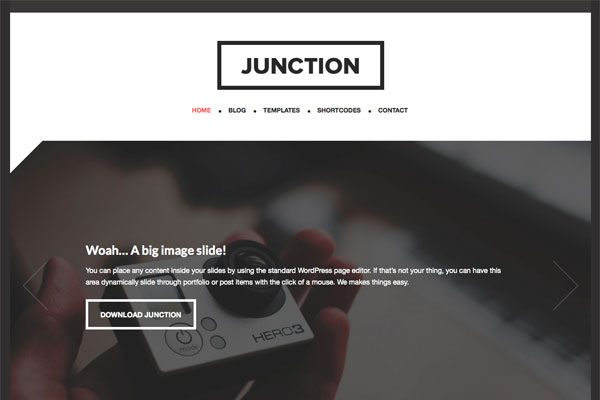The image captures a screenshot of a sleek, well-designed website, likely from a WordPress development suite. The top third of the image features a minimalistic header with the word "JUNCTION" in bold, black, all-caps text, encased in a black-bordered rectangle on a white background. Directly below this header is a five-option navigation menu with items labeled "Home" (highlighted in red), "Blog," "Templates," "Shortcodes," and "Contact."

The main section of the webpage prominently displays an alert message stating, "Whoa, a big image slide. You can place any content inside your slides by using the standard WordPress page editor. If that's not your thing, you can have this area dynamically slide through portfolio or post items with a click of a mouse. We make things easy." Below this message, there is a call-to-action button that reads, "Download JUNCTION."

Taking up the lower two-thirds of the image is a photograph of a human hand holding an electronic device labeled "Hero 3," which resembles a photography light meter or a guitar tuner. The backdrop behind this photograph is a subtle gray and white pattern, while faint navigation arrows flank the sides of the error message, indicating a slideshow feature for browsing images. The overall design is modern and user-friendly, suitable for dynamically displaying content.